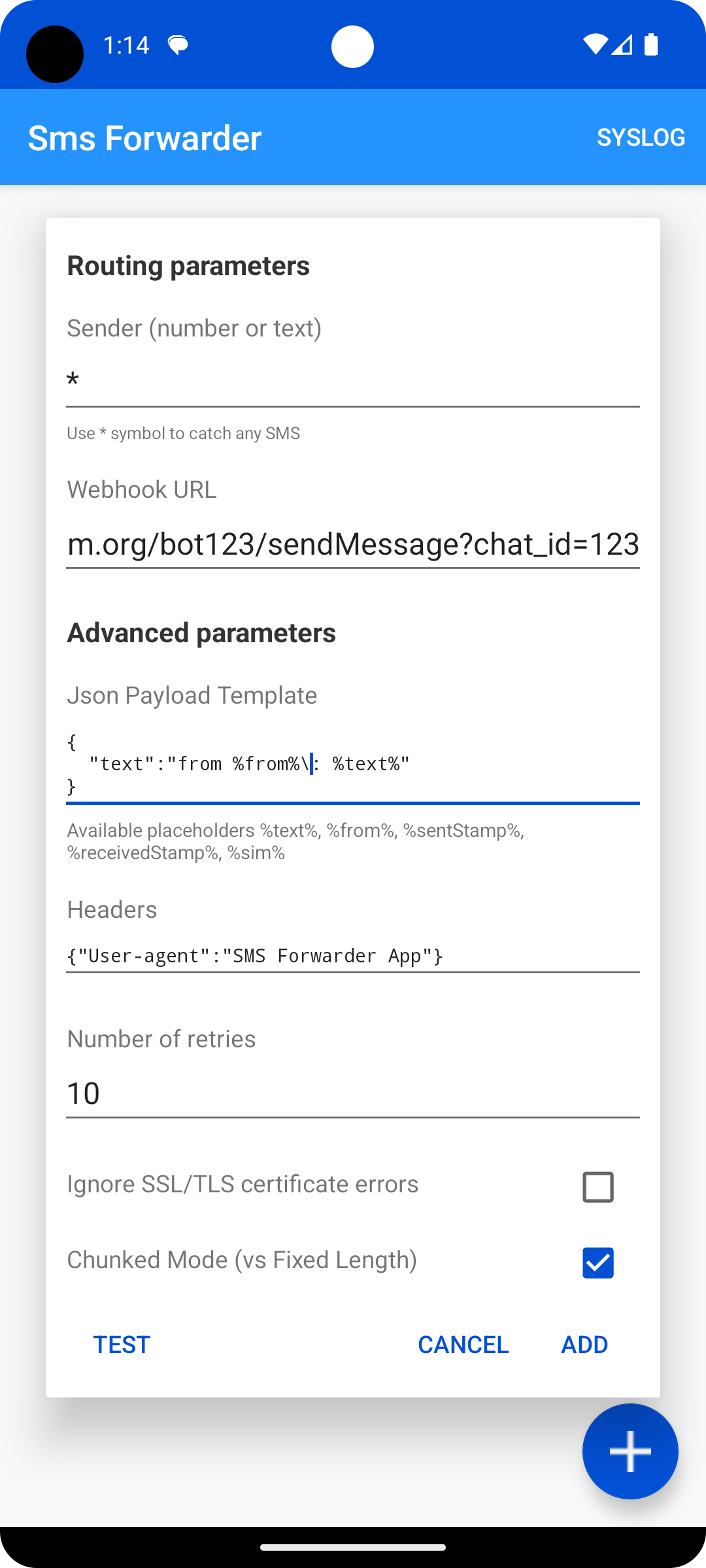The image is a mobile screenshot displaying the interface of an SMS forwarder app. At the top, there is a very thin blue status bar, followed by a slightly larger blue bar, both in a baby blue color. In the center of the screen, there is a white circle. Below this, the title "SMS Forwarder: Syslog" is visible.

Descending further, there is a white text box with black text that reads "Routing Parameters," followed by labels for "Sender," with a placeholder indicating "Number or Text." Below this label, there is an input field with a note that reads, "Use asterisk (*) symbol to catch any SMS." 

Further down, a labeled field "Webhook URL" is shown with the example URL "m.org/bot123/sendmessage?chat_id=123."

Beneath this section, the text "Advanced Parameters" is displayed, detailing more settings:

- "JSON Payload Template" followed by a complex placeholder: `{"text": "%text%", "from": "%from%"}`.
- A list of available placeholders: `text`, `from`, `sent_stamp`, `received_stamp`, and `sim`.
- "Headers" section specifying "User-Agent: SMS Forwarder App."
- "Number of Retries" is set to 10.

There are also configuration options with two checkboxes:
1. "Ignore SSL/TLS Certificate Errors"
2. "Chunked vs. Fixed Length" (the latter having a blue check mark).

At the bottom, there are three blue buttons labeled "Test," "Cancel," and "Add."